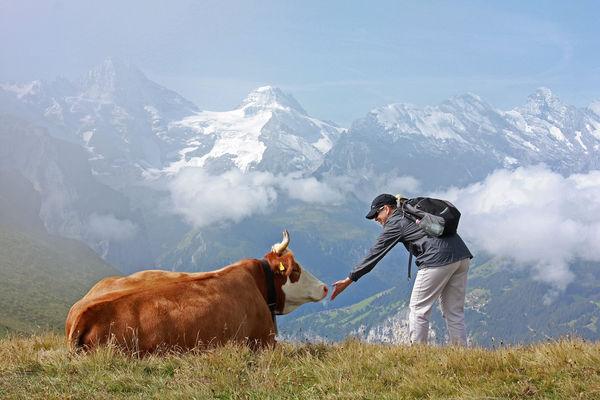In this detailed photograph taken from a high elevation, the setting is a grassy hill characterized by medium-length grass that is a mix of green, yellow, and orange hues. A woman, dressed in white slacks, a light gray jacket, a black and gray backpack, and a black hat, bends over towards the left side of the image. She is reaching her left hand towards a light brown cow with a white face and two small horns. The cow, adorned with a black collar and a yellow ear tag, appears to be sniffing her hand while lying on the patchy grass.

In the background, the scene is dominated by a panorama of towering, snow-capped mountains that rise above a blanket of clouds, giving the impression of being at an exceptionally high altitude. The mountains appear hazy and blurred due to the foggy or cloudy conditions. The overall atmosphere of the image is one of serene solitude and majestic natural beauty, encapsulating the high-altitude mountain landscape with its snow-laden peaks and expansive sky above.